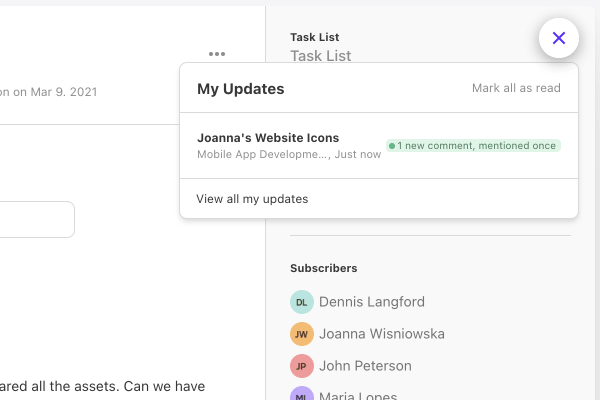This screenshot captures a detailed view of a computer screen displaying a task list, segmented into various sections. On the far right, there is a prominently labeled "Task List" column in black text. Directly below, "Task List" appears again, this time in a slightly larger and gray font. Beneath this repeated heading, a pop-up box emerges featuring a cancel icon in blue, encircled for emphasis.

Within the pop-up, the text reads: "My Updates: Mark All as Read," followed by "Joanna's Website Icons." Below that, the phrase "Mobile App Development - Just Now" appears, along with an indication of a new comment and a mention, denoted by a dot followed by "One New Comment, Mentioned Once." An option to "View All My Updates" sits at the bottom of the pop-up box.

Outside this pop-up, the right-hand column continues with a list of subscribers, including Dennis Langford (D.L.), Joanna Wisinowska (J.W.), John Peterson (J.P.), and Maria Lopez (M.L.). Each subscriber is identified with their initials encased in a colored circle.

On the left side of the screen, the date is clearly displayed as March 9th, 2021.